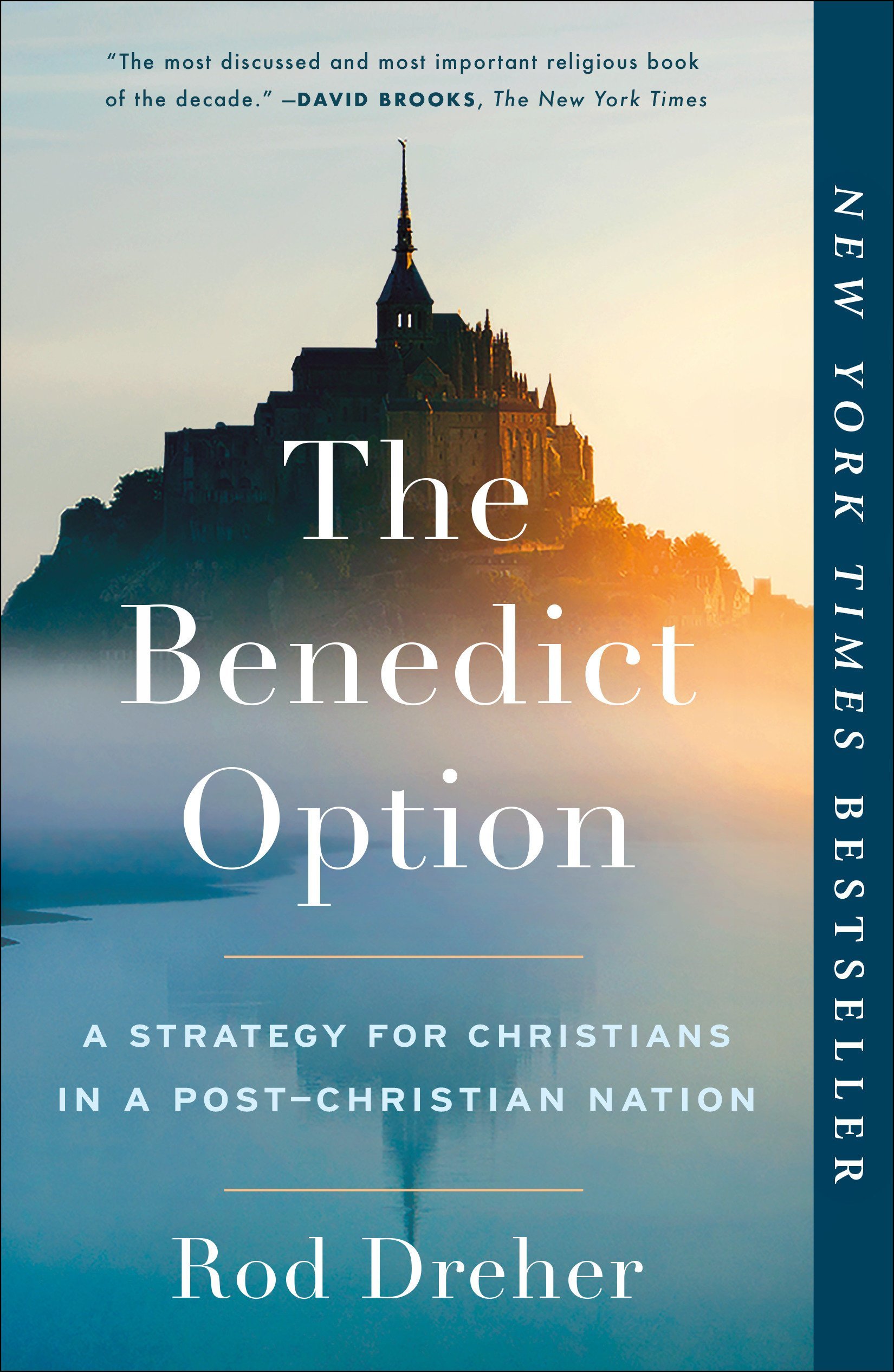This image is a detailed book cover. It features a vertically rectangular layout with a blue border running along the right side displaying "New York Times Best Seller" in white text. At the top, in small blue print, it states, "The most discussed and most important religious book of the decade," attributed to David Brooks of The New York Times. The central image depicts a majestic structure that combines elements of a castle and a grand church, perched atop a steep hill adorned with trees and rocks. The edifice, likely a monastery or cathedral, has a prominent spire and walls, reminiscent of medieval architecture. Below, the hill’s reflection can be seen in the calm, blue waters of a lake, with a thin line of fog hovering above the water. Overlaid on the image in white text is the book's title, "The Benedict Option," followed by the subtitle, "A Strategy for Christians in a Post-Christian Nation." The author, Rod Dreher, is credited at the bottom in white text. The composition of text and imagery together establishes a striking and significant visual appeal for the book cover.